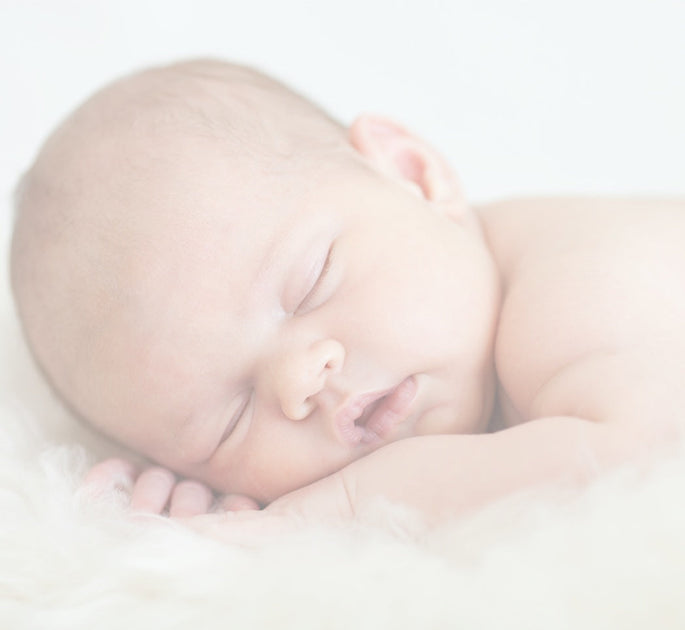The image is a square composition with predominantly skin tones and shades of gray. The focal point is a sleeping baby, who occupies the majority of the center space. The baby, likely newborn and Caucasian, is resting peacefully on a fluffy white substance that could be a blanket or pillow. The baby lies on its right side with chubby cheeks and closed eyes, suggesting contentment. Its mouth is slightly open, revealing red lips, and one ear is visible near the top of the image. The baby has fine, sparse dark hair, and its skin appears pale pink. One hand is tucked under the head, while the other rests in front of the face, showing tiny fingers. The image has a blurred, overexposed quality, giving it a dreamlike appearance. The background is plain white, offering no additional details or distractions.